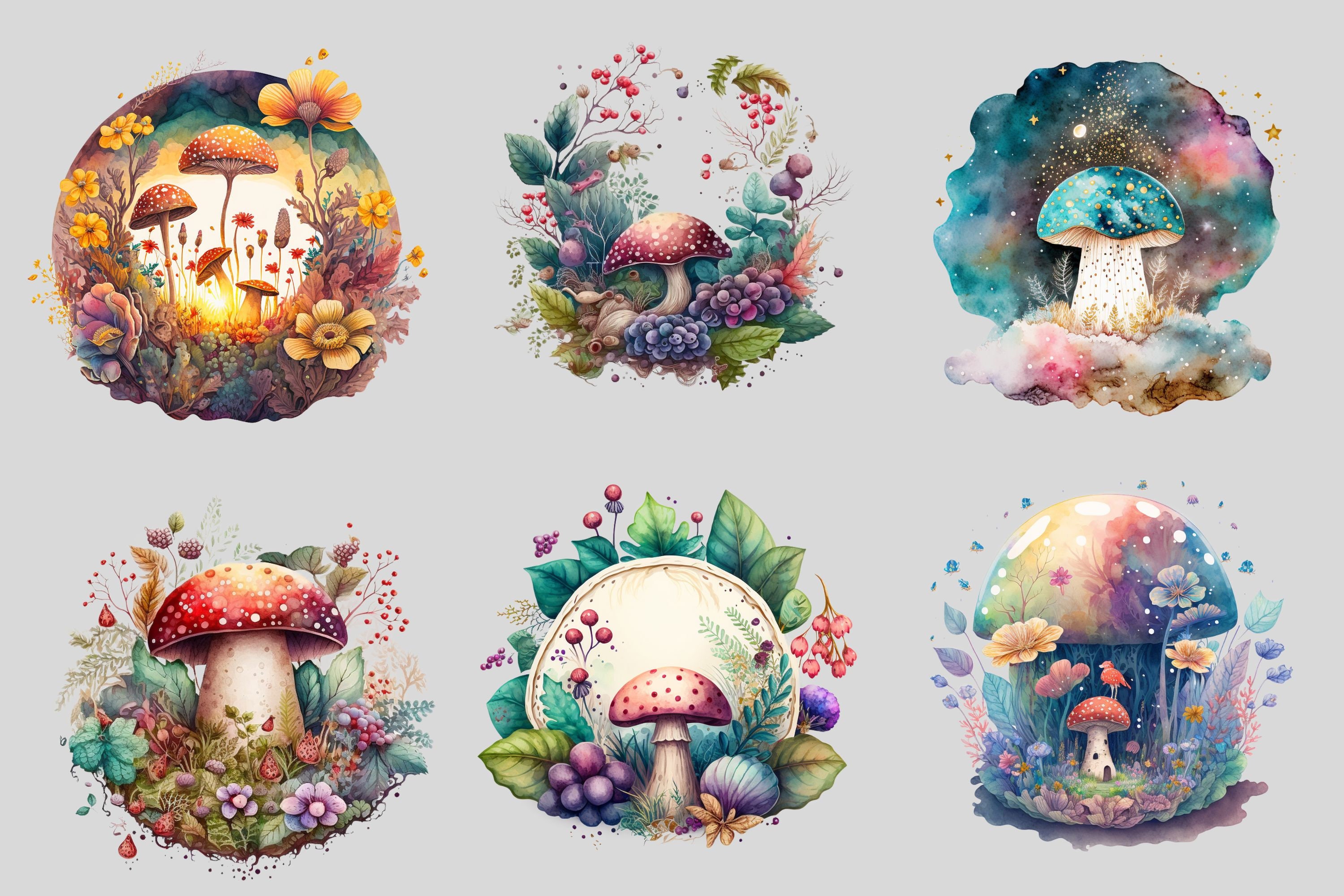The rectangular image with a gray background features six intricately designed and colorful illustrations of mushrooms, arranged in two rows of three. Each artwork centers around a mushroom, enveloped by various floral arrangements and unique scenic elements, crafted with vibrant, detailed aesthetics.

In the top row, the first image showcases four yellow mushrooms encircled by yellow and pink flowers, with a sunny, wreath-like design. The middle illustration depicts a white-stemmed mushroom with a reddish cap, set against a backdrop of blue flowers and leaves. The top right picture presents a psychedelic celestial scene featuring a white-stemmed, blue-capped mushroom with galaxy-like colors surrounding it.

On the bottom row, the first image displays a tall, thick mushroom with a white stem and red cap, surrounded by scattered flowers and leaves. The middle illustration portrays a red-capped, white-stemmed mushroom with what appear to be purple grapes and abundant leaves around it. The final image on the bottom right highlights a small red-capped, white-stemmed mushroom accompanied by a larger pastel-colored mushroom in the background, framed by an assortment of red, white, yellow, and blue flowers.

Each piece is distinctive yet unified by the theme of mushrooms and their natural, whimsical settings, reminiscent of art that could be found on platforms like Etsy or Pinterest.